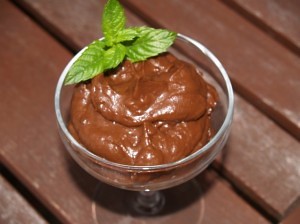This photograph captures a rich chocolate pudding, set in a clear glass shaped like a wine glass with a broad rim. The glass sits atop a brown wooden table or plank with diagonal paneling. The chocolate pudding exhibits a glossy texture, reflecting light subtly, implying a creamy and smooth consistency. Garnished on the pudding is a vibrant green sprig of mint, comprising about several leaves of varying sizes. The image is well-lit, shot from above, and shows no other objects, text, or dates, focusing solely on the delectable dessert against the rustic wooden backdrop.